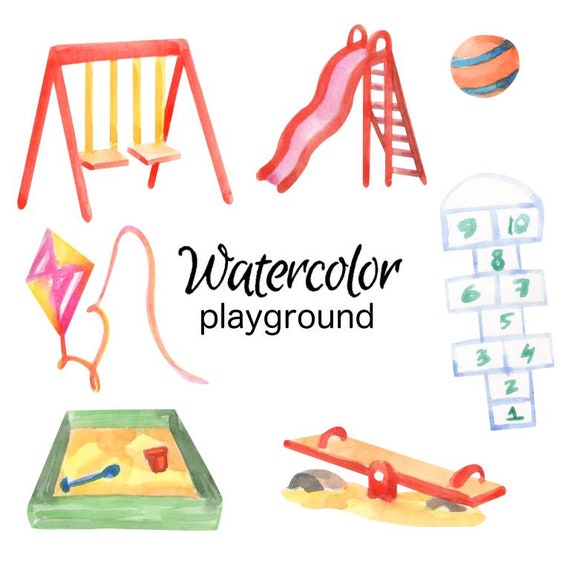This image is an illustration of a playful watercolor playground theme, with the central text "Watercolor Playground" in black on a white background, surrounded by various playground items. Starting from the top left, there's a red swing set with yellow swings. Right next to it is a red slide with hints of pink. Moving to the right, there's a light pastel orange ball with black and blue stripes. Beneath it is a colorful kite with red and yellow sections, followed by a hopscotch board featuring numbers one through nine in gray with green highlights. At the bottom left, there is a green sandbox filled with yellow sand, accompanied by a red bucket and a blue shovel. Lastly, in the bottom right, there is a red seesaw set in sand, tilted down towards the right.